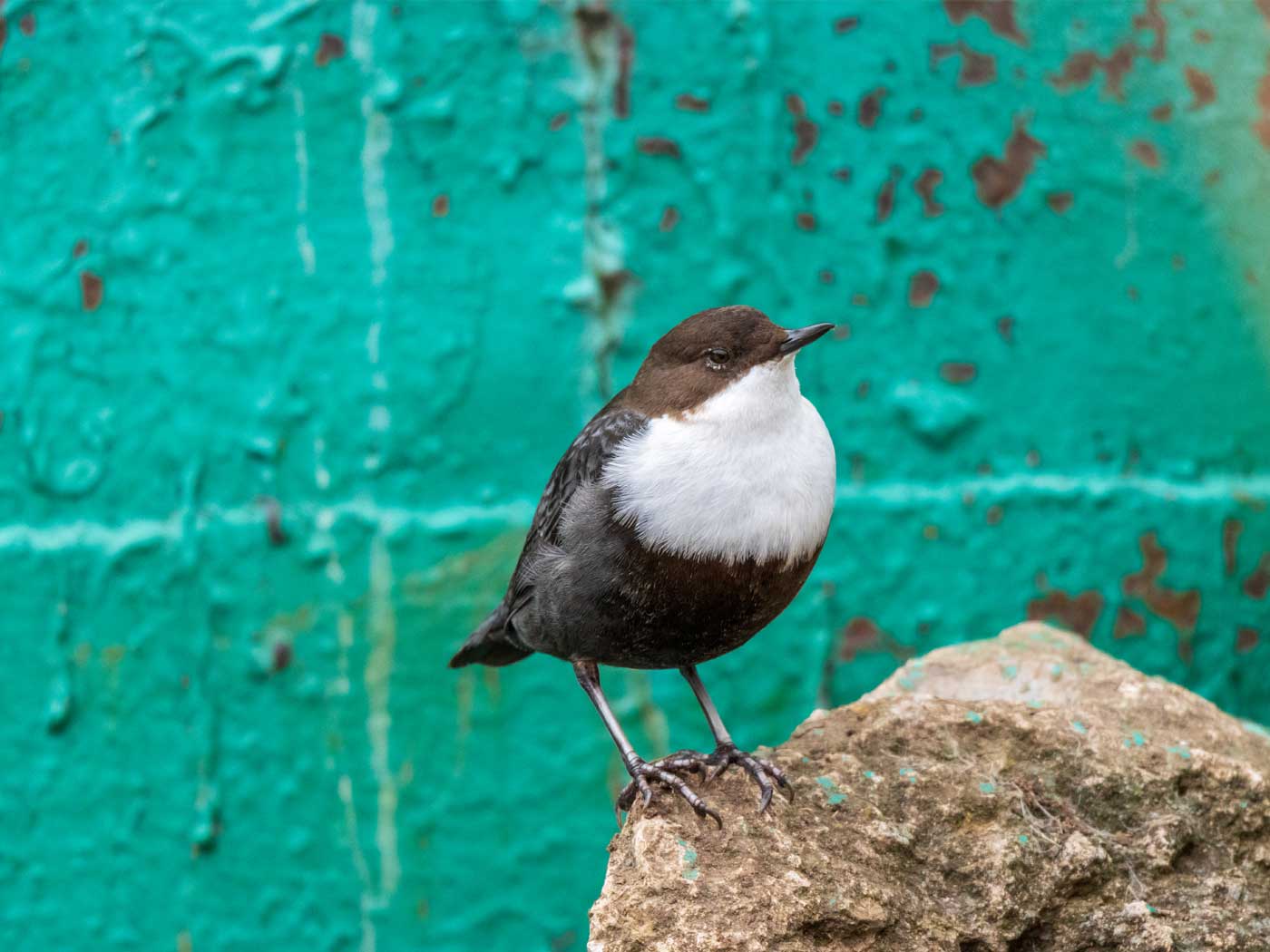In this highly detailed, close-up photograph, a small bird perches on a rough brown rock. The bird features a brown head, a black beak, and a white area covering its neck and upper chest, while its body and wings are predominantly black. The bird is centered and in sharp focus, revealing its intricate features, including its feet gripping the rock's edge. The background reveals an old, textured wall painted in a teal green or aqua blue color, which is peeling and cracking, exposing brown spots and white streaks beneath. Some areas of the wall show caked paint and dried run marks, enhancing its weathered appearance.